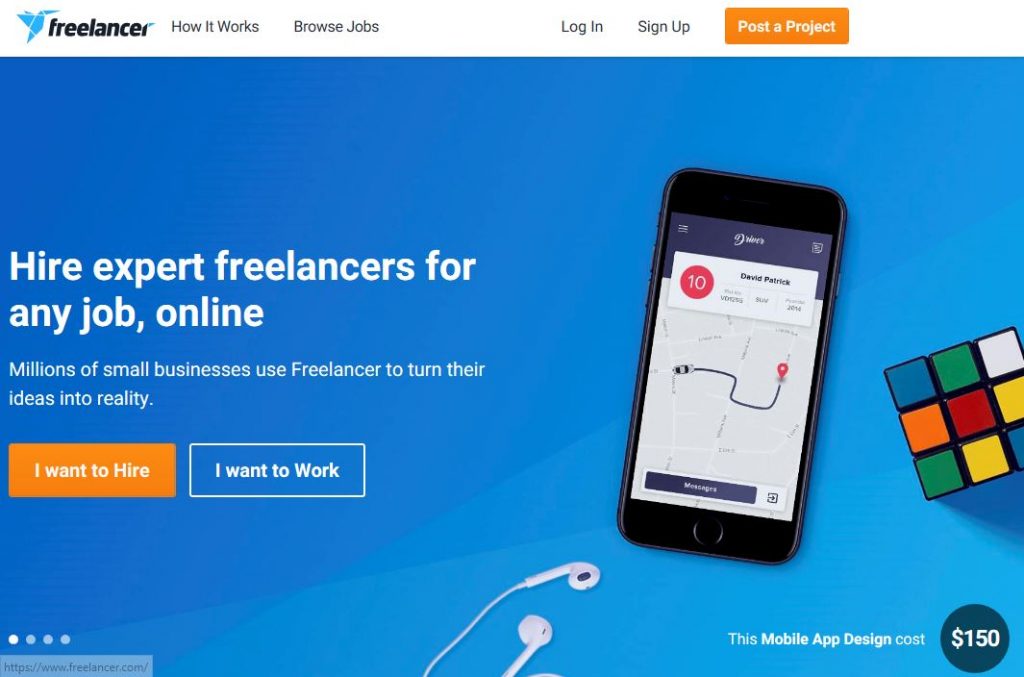This image showcases a website or an advertisement for a website, likely the homepage of Freelancer.com. The image is either in portrait or landscape orientation and does not have any defined outer borders. At the top, there's an icon resembling a blue origami bird followed by the word "Freelancer" in black font, with the tip of the 'R' in blue. 

Horizontal menu options appear next to the logo on a white background with black font, listing:

- How it Works
- Browse Jobs
- Log in
- Sign Up

Further to the right is an orange rectangular button with white text that says "Post a Project."

Beneath this header, a large blue box serves as the main background. This box is landscape in orientation, starting with dark blue at the top and gradually lightening as it descends. 

In the center-left of this blue background, prominent white text reads: "Hire expert freelancers for any job, online." Below it, smaller font adds, "Millions of small businesses use Freelancer to turn ideas into reality."

Two buttons are located within this section:

1. An orange rectangular button with white text saying "I want to hire."
2. A white rectangular button with white text saying "I want to work."

On the right side of the image is a picture of a cell phone displaying an app with the number "10" on the screen. Adjacent to the phone is a Rubik's Cube. At the bottom of the image, a partial picture of headphones is visible. Above these items, text indicates "This mobile app design cost," alongside a dark blue bubble with the number "150" in white inside it.